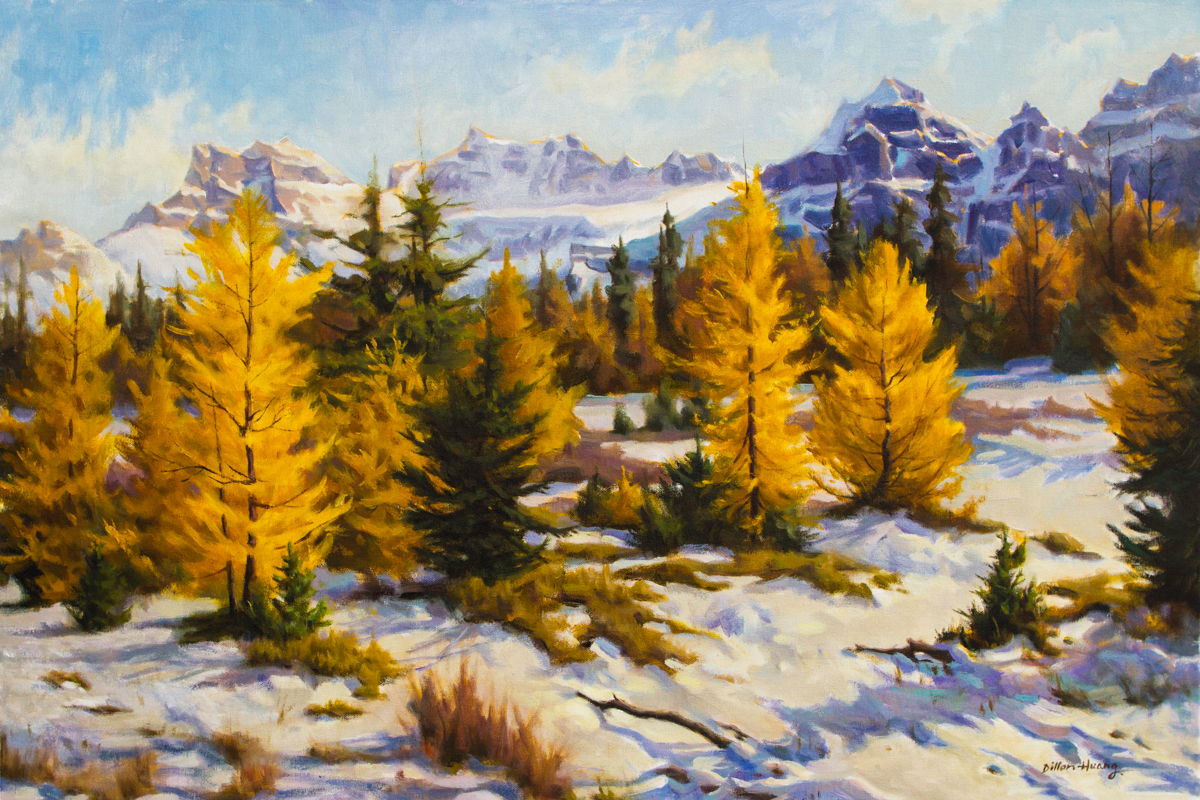This painting depicts a tranquil outdoor scene set against a mountainous backdrop. The foreground features a snow-covered expanse, dotted with scattered sticks and bushes emerging through the snow. Throughout the middle of the image, a mixture of green and yellow pine and fir trees can be seen, varying in size from small, young saplings to taller, more mature trees. These trees are dispersed from left to right, creating a natural, uneven row. In the background, another stand of similarly colored trees stretches across the scene, leading up to imposing brown mountain peaks. The peaks are blanketed with patches of snow, and the sky above is a blend of blurry blue and white, suggesting clouds. The entire landscape is bathed in soft sunlight, casting gentle shadows across the snow-covered ground. The artistic style, possibly watercolor or oil-based, lends a serene and almost ethereal quality to the scene, reminiscent of a peaceful winter day in the Colorado hills.